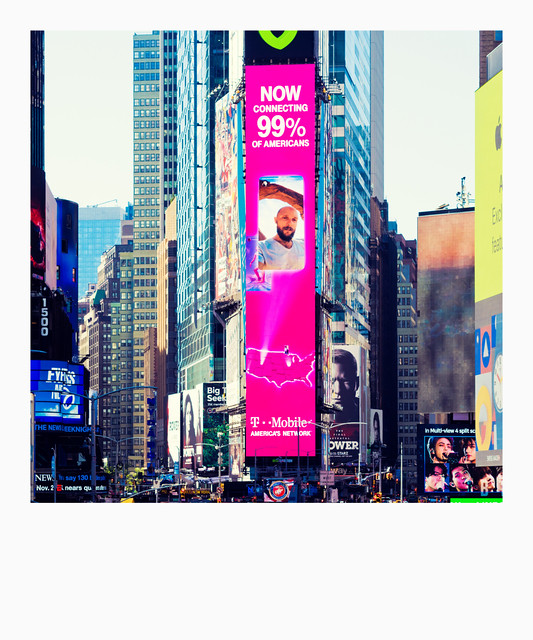The image depicts a bustling Times Square scene in downtown New York City, characterized by its towering high-rise buildings adorned with numerous vibrant billboards. Dominating the center is a striking, vertical T-Mobile advertisement, notable for its bright Barbie-pink color. This eye-catching billboard features white text that reads "Now Connecting 99% of Americans," alongside a picture of a bald man with a beard standing outdoors, with a tree branch visible behind him. Below the text is an outlined map of the United States, highlighted with illuminated areas, and at the bottom, it states "T-Mobile America's Network". The photograph captures a daytime, slightly overcast sky, with additional billboards visible on adjacent buildings and a bustling ground level with elements such as possible taxicabs, people, and activity indicative of New York's vibrant street life. In the bottom left corner, the word "news" is visible, while on the lower right, a group of people appears to be singing into microphones. The scene portrays the dynamic and unmistakably busy atmosphere of Times Square.